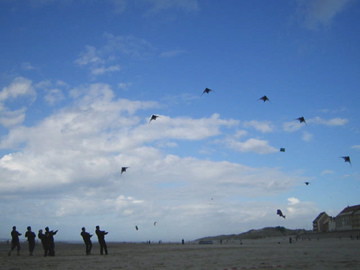The image captures a vibrant outdoor scene on what appears to be a delightful day. Dominating the composition is a bright blue sky, mostly clear but punctuated by a few white, puffy clouds. The sky takes up about 90% of the image, creating a sense of openness and vastness. In the bottom left corner, six people are clustered together, likely engaged with the ten kites that are soaring in the sky. The kites, which could be mistaken for fighter jets or birds due to their shapes and the way they are flown, create dynamic patterns, forming a circle as they fly outward. On the bottom right corner, a house is visible, accompanied by a grassy hill, adding a touch of quaint charm to the scene. The people, appearing to guide the kites with strings, are dressed in dark clothing, standing out against the bright landscape. Overall, the image beautifully captures the joy and simplicity of kite flying on a picturesque day.